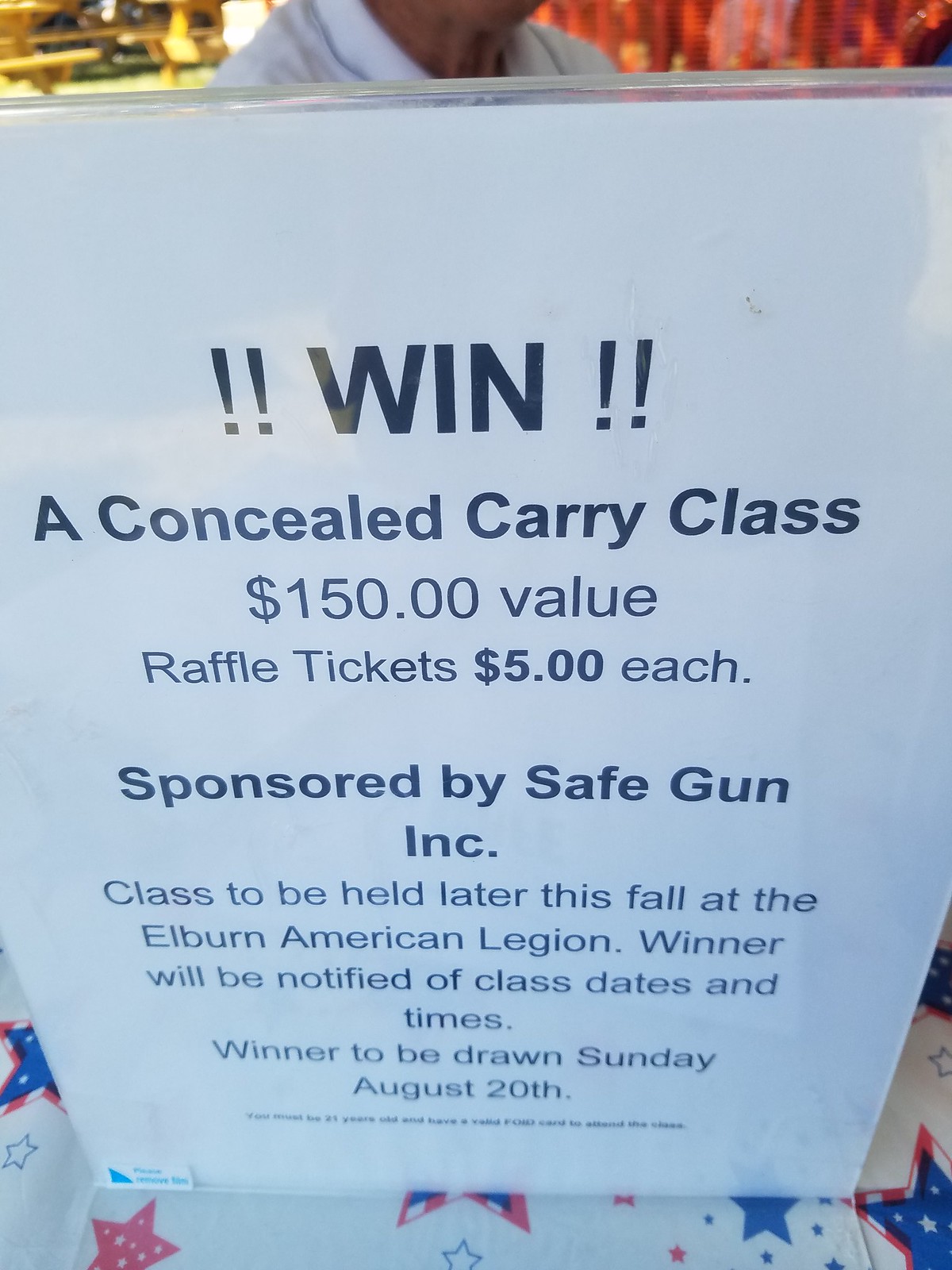The image captures a vibrant scene at what seems to be an outdoor event, possibly a farm fair. Central to the photograph is a sign encased in a plastic frame, prominently placed on a table covered with a patriotic red, white, and blue star-patterned tablecloth. The sign, which is printed on white paper with black text, announces a raffle: "WIN!! A concealed carry class, $150 value. Raffle tickets $5 each. Sponsored by Safe Gun Inc. Class to be held later this fall at the Elburn American Legion. Winner will be notified of class dates and times. Winner to be drawn Sunday, August 20th." At the bottom, there's a line of small, nearly illegible print, likely containing additional terms or disclaimers. In the background, the neck and shoulders of an older person in a white polo shirt are visible, along with several tables set up in the distance, hinting at the bustling atmosphere of the event.